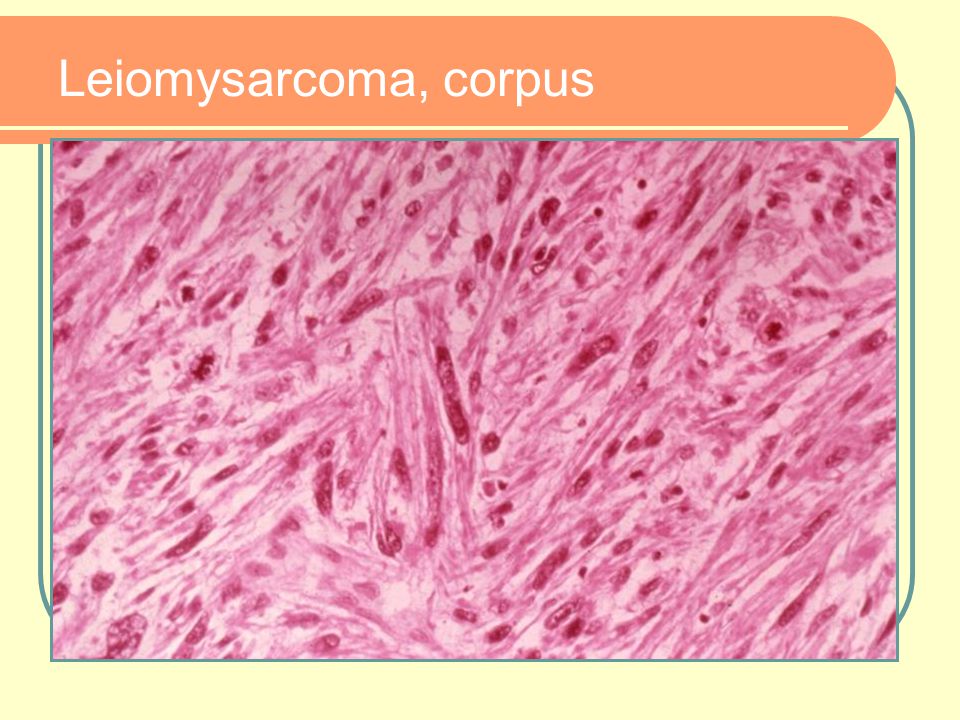The PowerPoint slide features an orange banner at the top, with white text displaying the title "Leiomysarcoma Corpus," spelled as "l-e-i-o-m-y-s-a-r-c-o-m-a space c-o-r-p-u-s," with only the initial 'L' capitalized. Below this banner is a detailed microscopic image of cells, predominantly filled with shades of pink, white, and red, exhibiting a complex, interesting pattern with numerous lines intersecting at various angles. The image has a green border and is set against a light yellow background, with a green line seamlessly connecting the orange banner to the image, providing a cohesive and visually structured layout.